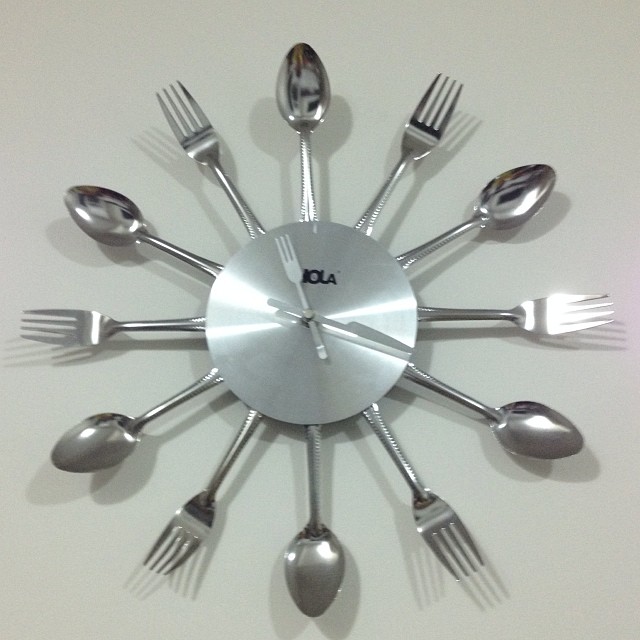The photo depicts an eccentric and unique analog clock, creatively crafted from shiny silverware. Mounted on a white wall, the clock features an outer ring composed of alternating silver forks and spoons, totaling 12 pieces, with spoons positioned at the 12, 2, 4, 6, 8, and 10 o'clock marks, and forks at the 1, 3, 5, 7, 9, and 11 spots. At its center, a silver circular disc serves as the clock face, adorned with two hands: a white fork indicating the hour and a white knife pointing the minutes. Near the top of the disc, partially obscured, there's black text that appears to say "Nola." The clock hands show a time of approximately 11:20. The silverware elements catch and reflect light, suggesting a light source directly above, adding a touch of sparkle to this whimsical timepiece.